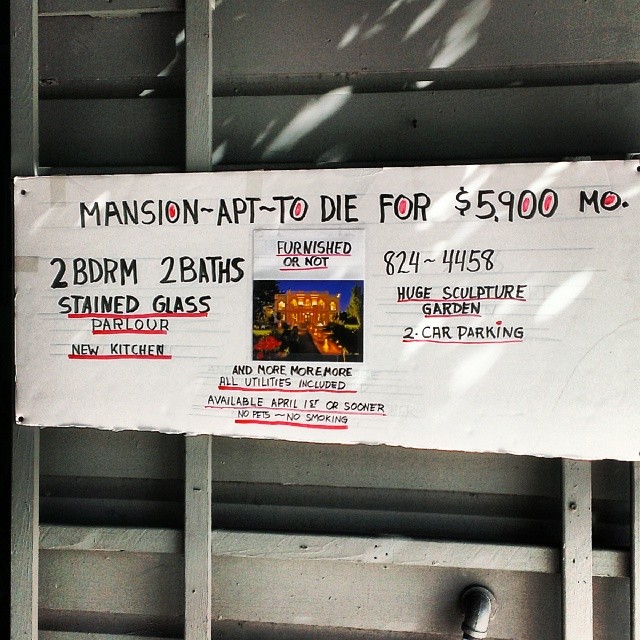This image features a handwritten advertisement for a rental property, posted on a wall composed of gray wooden slats. The sign itself is a horizontal white piece of paper with text and a photograph of a beautifully lit mansion at night in the center. The advertisement reads: "Mansion apt to die for, $5,900 a month. Two bedrooms, two baths, stained-glass parlor, new kitchen, furnished or not, and more, more, more. All utilities included. Available April 1st or sooner. No pets. No smoking." To the right of the mansion photograph, the contact phone number 824-4458 is displayed. Additional highlights include a huge sculpture garden and two-car parking. Despite the luxurious description, the advertisement appears surprisingly low-quality, which juxtaposes the high-end nature of the rental property it describes.